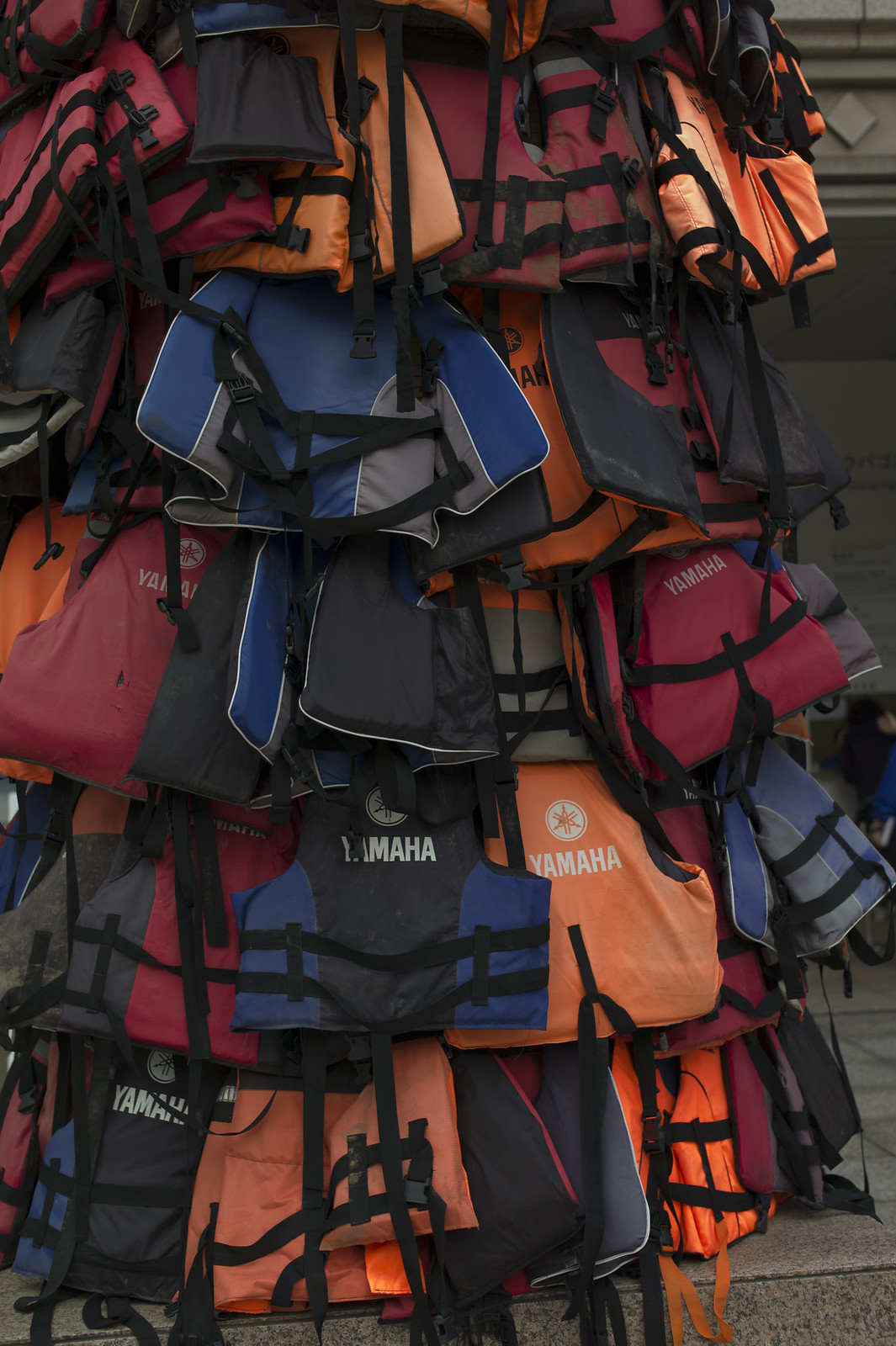The photograph depicts a large collection of Yamaha-branded life jackets hanging from a metal, tree-like structure. The vests are in various states of use, some with noticeable sand and dirt. They come in a range of colors including bright orange, red, black, and blue. Each life jacket features straps and buckles essential for ensuring a snug fit. The Yamaha logo, a circle with a six-pointed star, is visible on many of them. The life jackets are neatly organized, suspended from the frame rather than piled on the ground, creating an almost overwhelming visual of dozens of flotation devices meant for safety on the water.